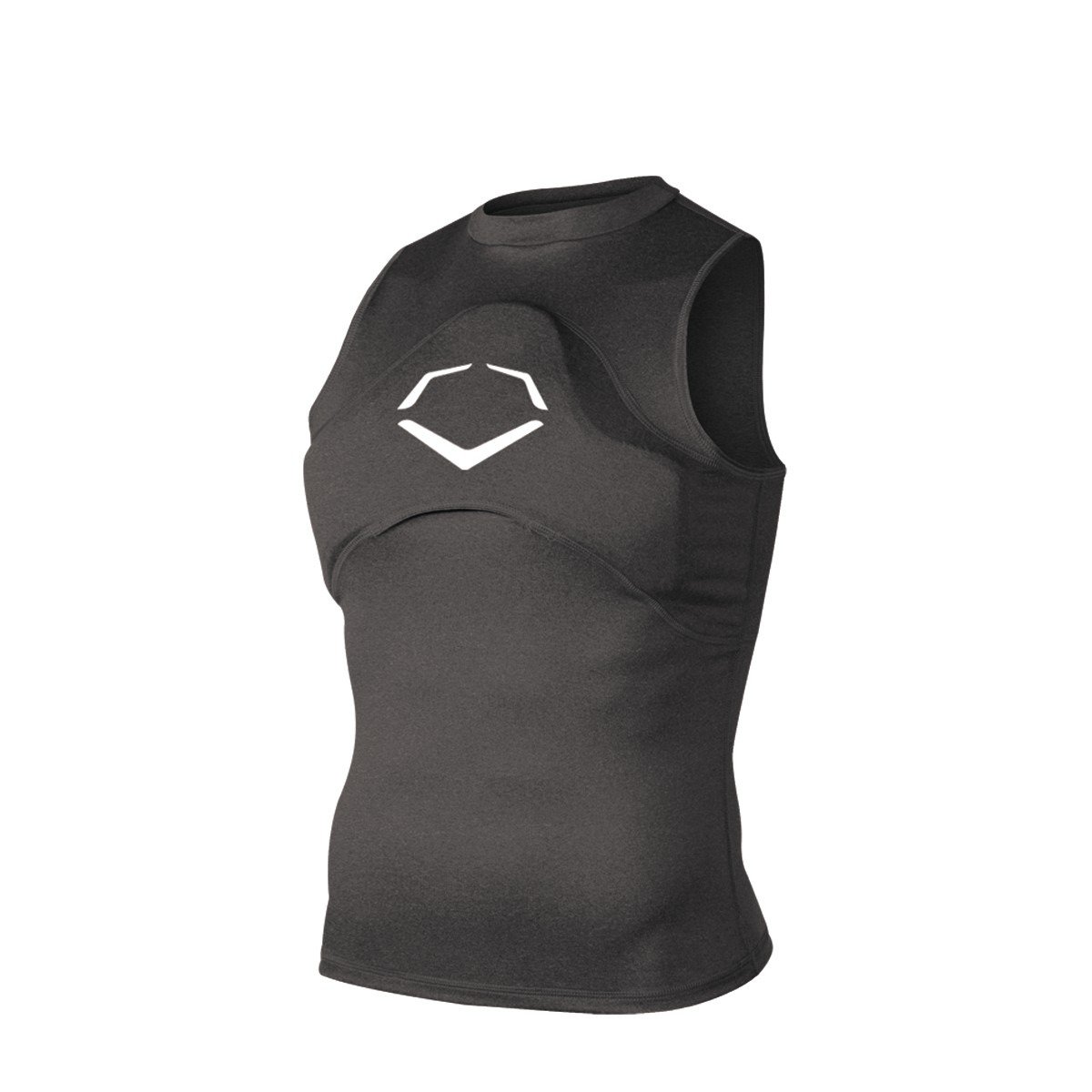The image features a close-up of a sleek, black, sleeveless sports top designed for either men or women, commonly found on shopping platforms like Amazon or company websites. The top is form-fitting, similar to body armor or a wetsuit but notably thinner. It features an arch-shaped padded section that starts below the neck, extends underneath the arms, and loops back up and down, providing enhanced chest support. This padding is under the fabric but visibly stands out from the rest of the garment, indicating its reinforced nature. Centered on the chest padding is a distinctive white logo, comprising an inverted V flanked by two horizontal lines, making a striking angular design. The top is showcased on a plain white background, emphasizing its contours and detailing for potential buyers.